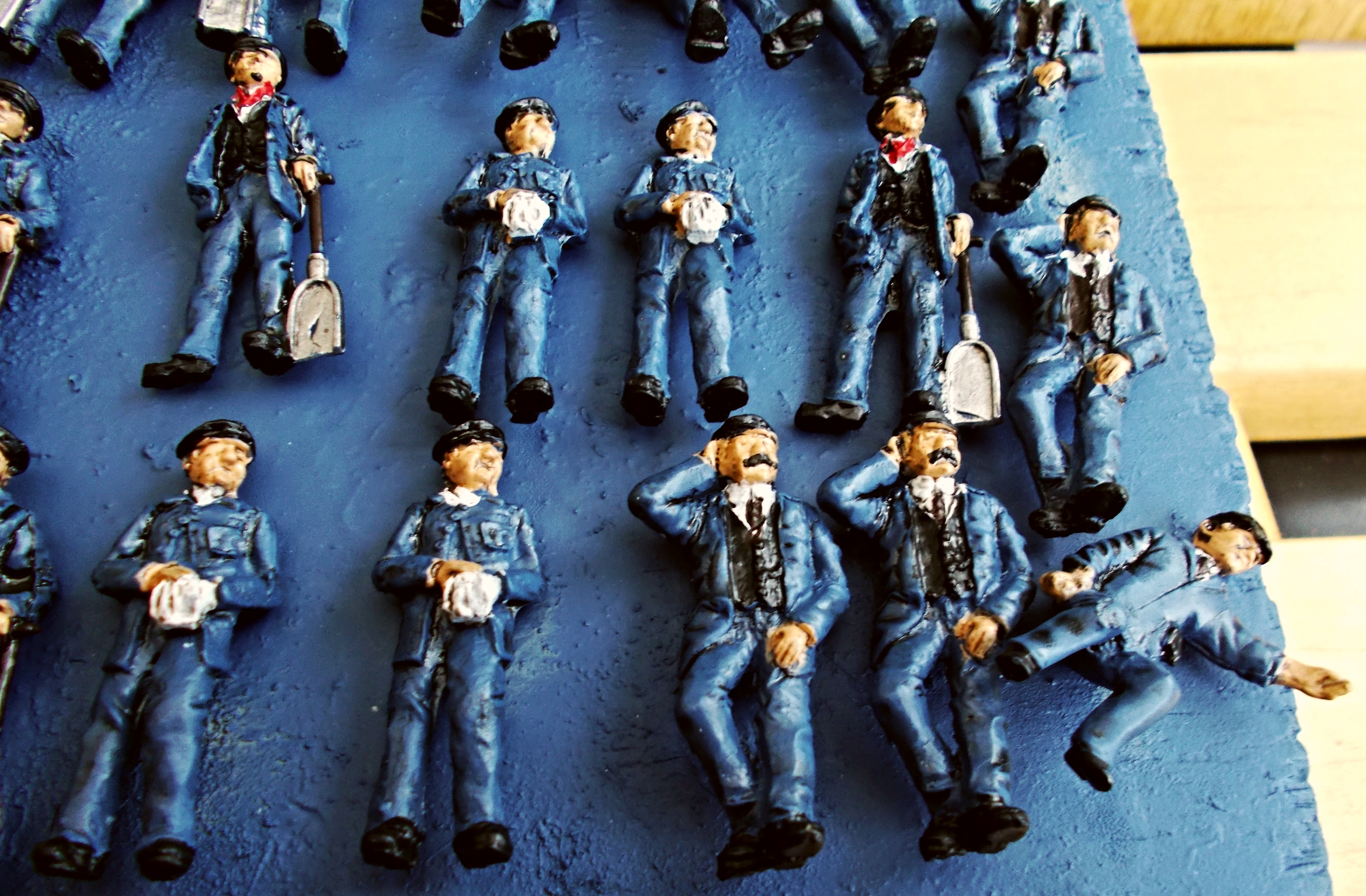In this detailed photograph, we see an assortment of custom-made action figures spread across a textured blue painted surface, possibly a concrete table with wooden panels visible to the right. Organized into at least three distinct rows, each figurine is dressed uniformly in blue long-sleeve shirts, matching pants, black vests, and white collared shirts, finished with black shoes. They all sport a black hat with a flat brim reminiscent of a police officer's cap. The figurines exhibit slight variations: some have a mustache, others are clean-shaven; several hold shovels, while a few grasp a white cloth or napkin. Certain figures adopt different postures; for instance, one has their hands folded, two have their left hand in their pocket with their right hand raised to their head. This curated array of figures, uniform yet unique in their minor differences, creates an intriguing and engaging visual.